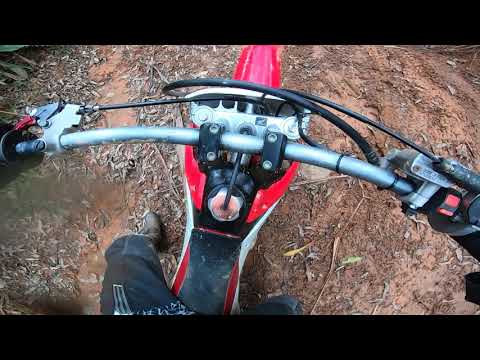This color photograph, captured from a GoPro, offers an immersive point-of-view shot as if from the top of the rider's helmet. It captures the moment a rider is situated on a mountain bike, indicated by the distinct red body and black footrest. The rider's gloved hands rest on the curved, unpainted steel handlebars, which are slightly cut off in the image, with visible brake levers on both sides. The rider appears to be wearing black trousers with graphic prints and brown boots, visible from knee to foot. The scene is set on a dirt path, strewn with sticks, branches, and gravel, creating a rugged terrain. The photograph, framed by black rectangles at the top and bottom, emphasizes the gritty environment interspersed with sparse vegetation. This detailed freeze-frame from a GoPro captures the essence of the rider’s adventurous spirit on a rugged dirt trail.